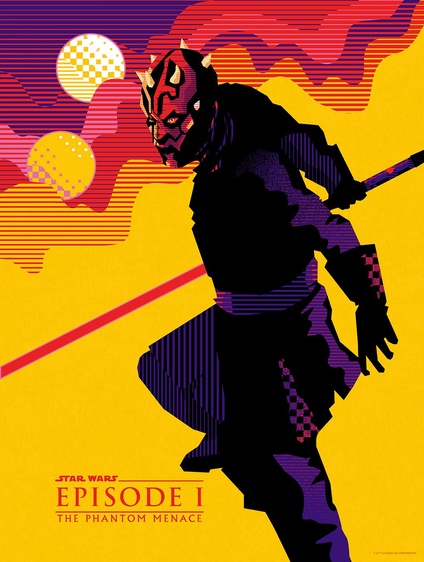This detailed movie poster for *Star Wars Episode I: The Phantom Menace* prominently features the menacing figure of Darth Maul in an action pose. He wields a red lightsaber in his right hand, with his legs bent and stretched to one side, demonstrating agility and power. Darth Maul's striking appearance is highlighted by his red and black facial markings and menacing yellow eyes, with red spikes protruding from his head.

Set against a vibrant yellow background that extends from the bottom left to the top right corner, the poster also includes hues of purple, pink, orange, and red, creating a dynamic and colorful scene. These colors form wavy and striped patterns across the backdrop. Two moons or circles, one yellow and one white with orange tinges, are visible in the upper part of the image, adding an otherworldly feel.

The text "Star Wars" appears in bold red letters at the top, with "Episode I" below it in capital red letters of a smaller font size, and "The Phantom Menace" in even smaller red letters underneath. Darth Maul is depicted wearing a black jacket with black gloves that show hints of purple in a checker pattern, adding depth and texture to his ominous presence.